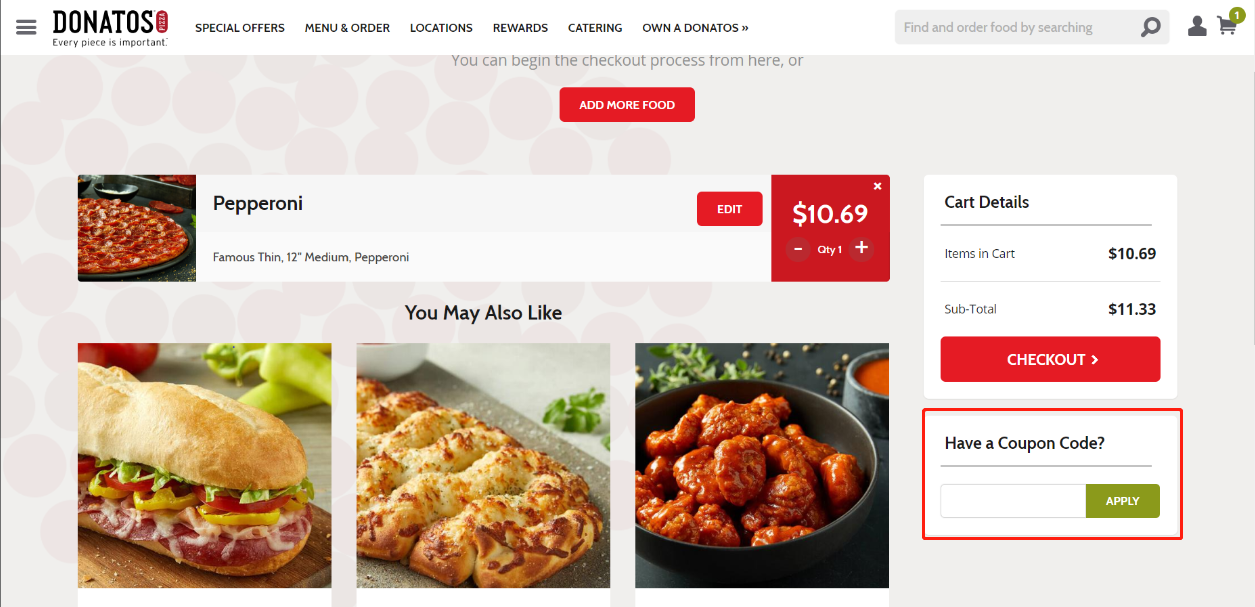The webpage belongs to Donato's, an Italian pizza restaurant, and displays the checkout section for an order. The focal point is a 12-inch medium thin crust pepperoni pizza, priced at $10.69 and highlighted within a red box. Adjacent to this, there's a "You May Also Like" section featuring three images of additional food items: a sandwich, a cheese bread, and a serving of wings.

To the right, detailed cart information is visible, itemizing the current order and costs. The pepperoni pizza costs $10.69, leading to a subtotal of $11.33, with a prominent red checkout button below. Underneath, there's a coupon code input area with a prompt that reads "Have a coupon code?" and a green "Apply" button next to it.

At the top of the page, several navigational tabs are present: Special Offers, Menu & Order, Locations, Rewards, Catering, and Own a Donato's. To the right of these tabs, a search icon, a profile icon, and a cart icon with a green circle bearing the number "1" are displayed, indicating one item in the cart.